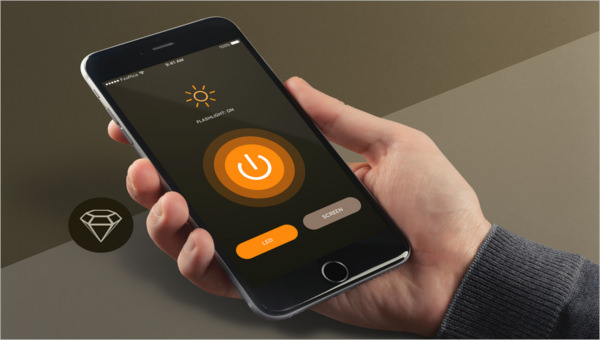In the image, a hand wearing a gray sweater holds an iPhone against a tan backdrop. The phone displays a screen with a sun icon at the top, followed by a prominent, orange power button encircled by various shades of orange rings. Below this power button are two additional buttons, one orange and the other gray, although the text on these buttons is blurry. A distinctive white diamond outline is located in a circle towards the bottom left of the screen. The iPhone is held in the right hand, possibly near a table surface.